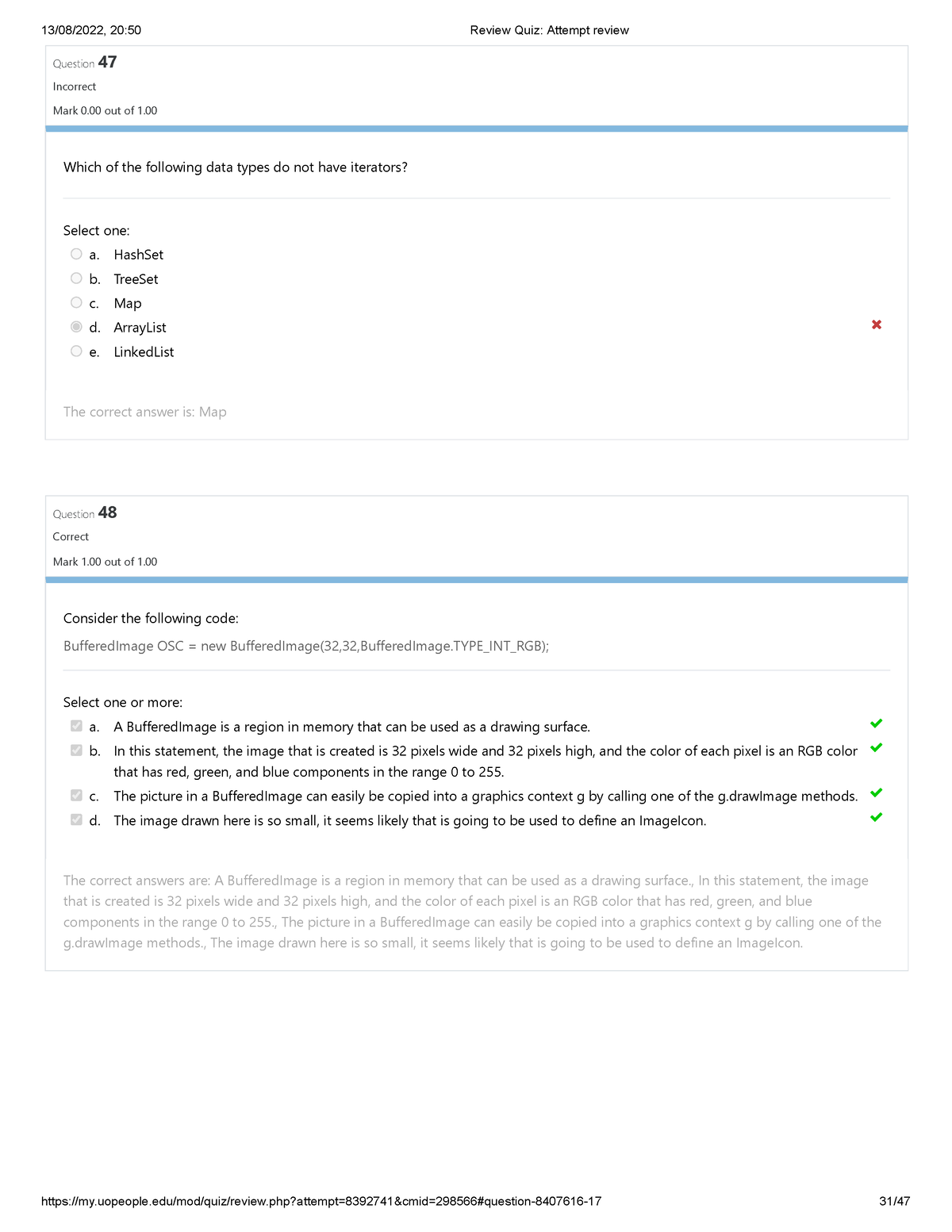At the top of the image, there is a date formatted as "13/08/2022." To the right of the date, "20.50" is displayed. On the same line, it says "Review Quiz Attempt 2." Below that, there is a block section labeled "Question 47." This section indicates that the question was answered incorrectly. It is marked with a score of "0.00 out of 100." A thin blue line separates this information from the question itself.

The question posed is: "Which of the following data types do not have Iterators?" This is a multiple-choice question with the following options:
1. HashSet
2. TreeSet
3. Map
4. ArrayList
5. LinkedList

The correct answer highlighted is: Map.

Following this, there is another block labeled "Question 48," showing that this question was answered correctly. The text begins with, "Consider the following code," followed by a line of code and various possible answers. The specifics of the question and answer options are partially obscured.